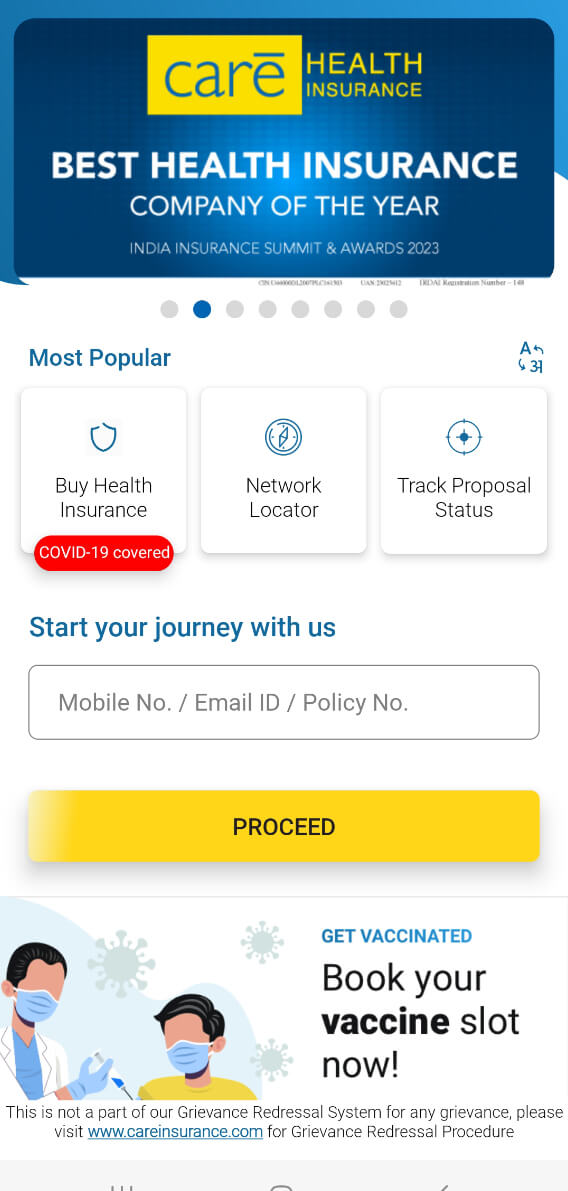Image Description:

The image captures a mobile website for Care Health Insurance. The website design indicates it might also function as an app, as there is no visible navigation bar at the top, possibly due to the user having scrolled down the page.

At the top, a large banner prominently displays the Care Health Insurance logo, affirming its identity. This is the second banner in an eight-panel slideshow, which includes the following text: "Care Health Insurance - Best Health Insurance Company of the Year, India Insurance Summit and Awards 2023."

Below the banner is a section titled "Most Popular," showcasing the top search categories:
- Buy Health Insurance
- Network Locator
- Track Proposal Status
- COVID-19 Covered (highlighted in a red, emergency-like color)

This is followed by a call-to-action section encouraging users to "Start Your Journey with Us." Here, users can enter their mobile number, email ID, or policy number into clearly marked input boxes before proceeding further.

At the bottom, there is an illustration featuring a doctor administering a vaccination shot to a masked man. A call-to-action below the illustration reads: "Get Vaccinated - Book Your Vaccine Slot Now."

At the very bottom of the page, a note clarifies: "This is not part of our grievance redressal system. For any grievance please visit careinsurance.com for the grievance redressal procedure."